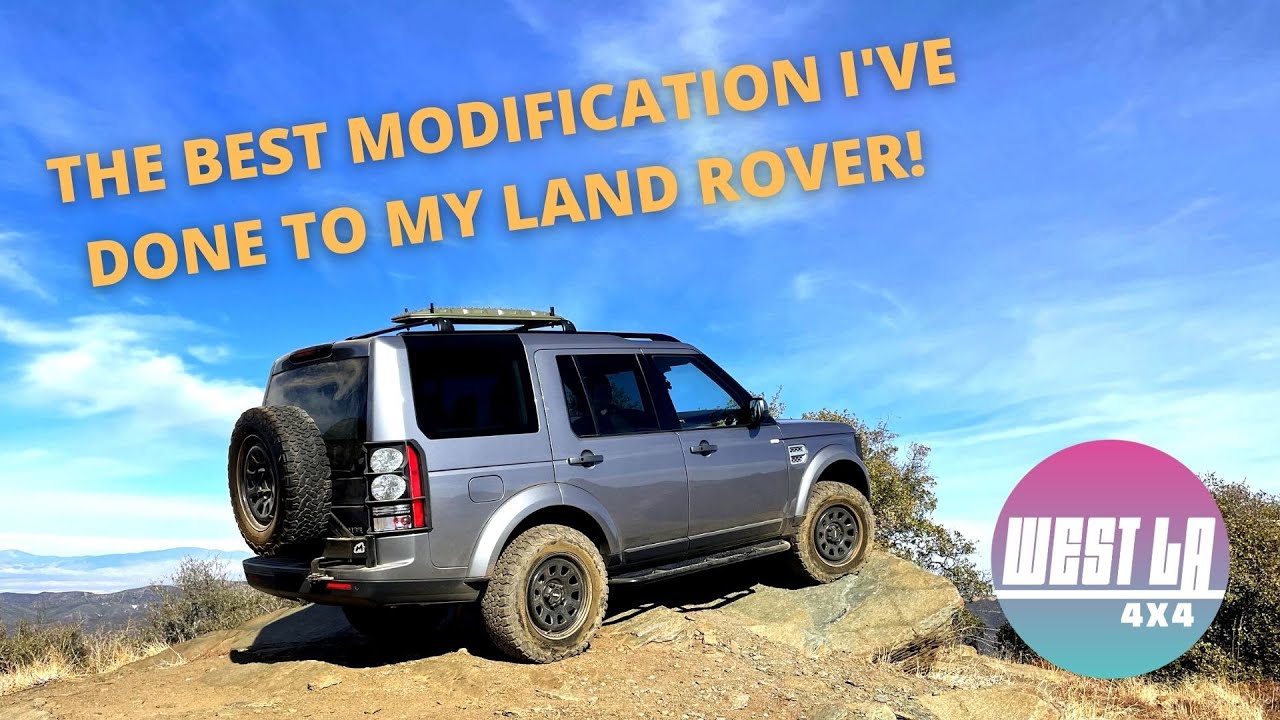In this edited image, likely sourced from social media or an advertisement, a gray Land Rover with black-tinted windows is prominently featured. The vehicle, shown from a side angle that highlights its right side, is perched atop a rocky cliff, indicative of off-road use. The tires, which are notably dirty, suggest recent rugged terrain navigation. The backdrop showcases a vibrant blue sky and distant mountainous scenery, adding depth to the visual. Key text in bold, yellow all-caps reads, "The best modification I've done to my Land Rover," suggesting a testimonial or endorsement. Additionally, the bottom right corner bears a purple-and-blue emblem for West LA 4X4, reinforcing the off-road adventure theme.